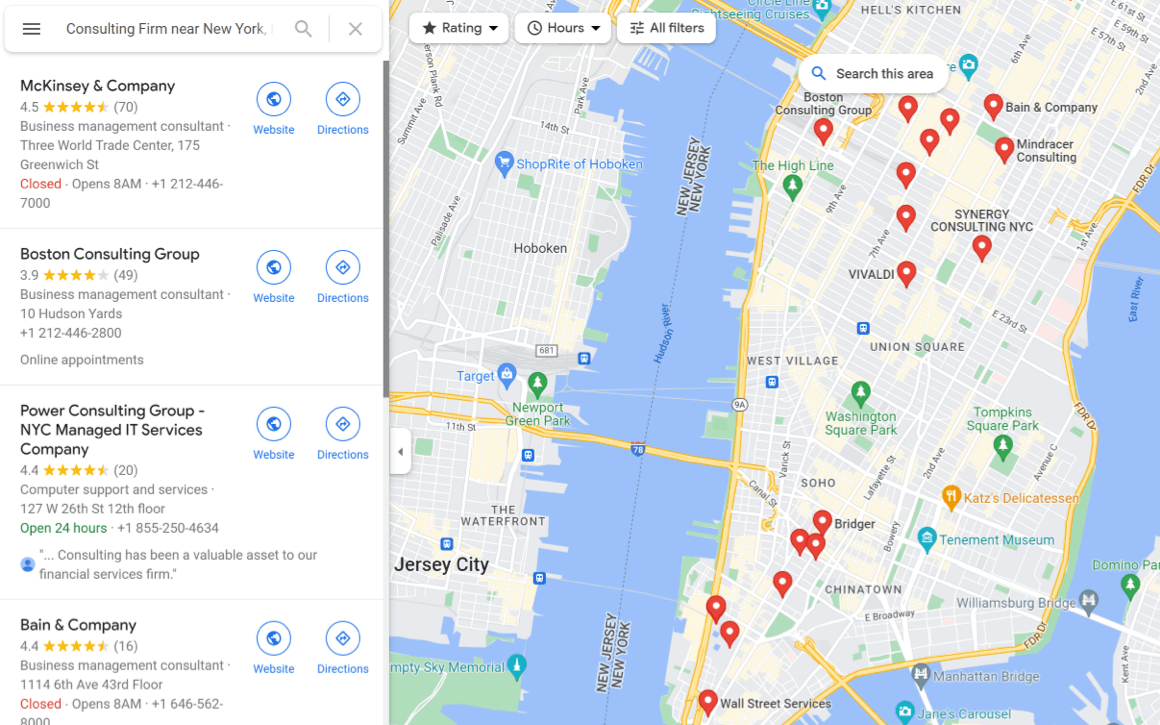This image is a screenshot from Google Maps, showcasing the search results for "Consulting Firm, New York." The screenshot is in landscape orientation and has proportions similar to a computer monitor display. 

On the left side of the image, there's a vertical white box listing search results for consulting firms. At the top of this box, there is a search bar with a hamburger menu icon to the left, followed by the search query in bold black text. Beneath this are various consulting firms listed with their names, star ratings, website links, and directions icons in blue. The firms include McKinsey & Company, Boston Consulting Group, Power Consulting Group, and Bain & Company, all of which have ratings close to four stars or higher.

To the right of the search results is a square-shaped map. This map displays the region around the New Jersey-New York border. The map highlights an area with bodies of water, likely the Hudson River, with numerous search results indicated by red pinpoints. Key locations on the map include parts of New York City, such as the West Village, and neighboring areas in New Jersey, including Hoboken and other identifiable landmarks.

Overall, the screenshot effectively splits the information into two sections: the detailed search results on the left and the geographical map representation on the right.